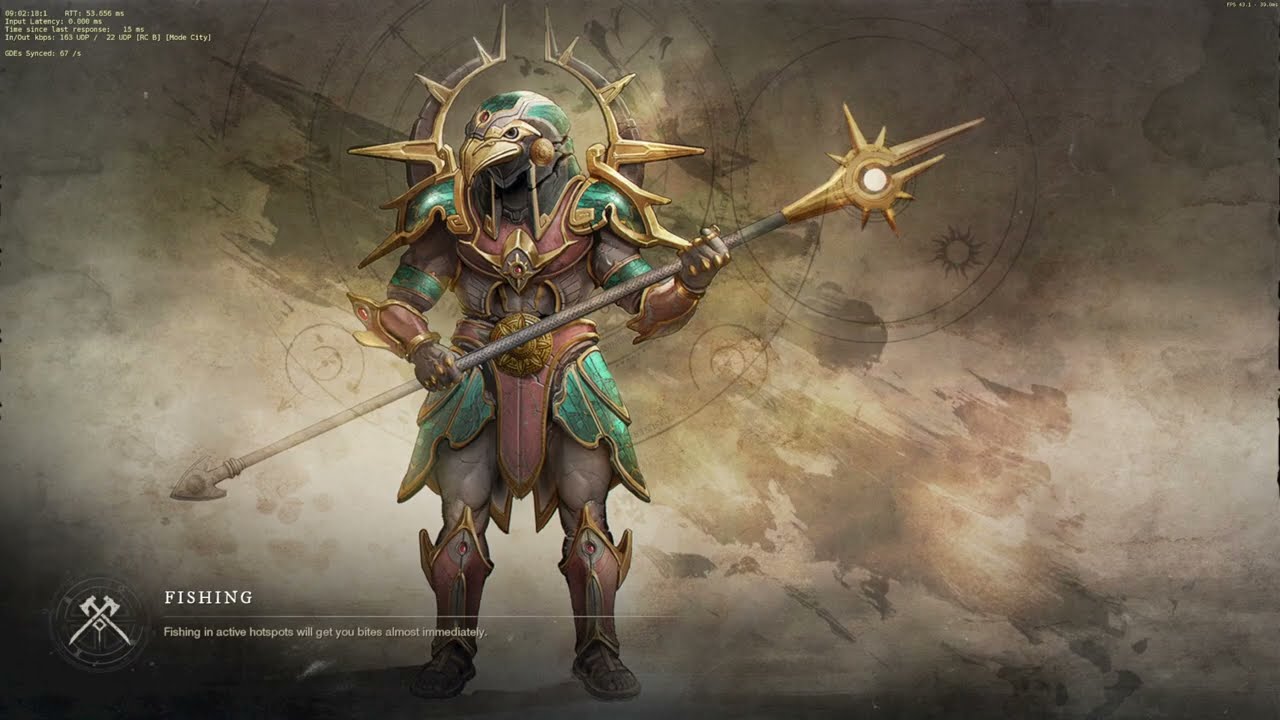In this wide rectangular digital artwork or video game character image, the background features a grayish light tan color resembling damaged paper, adorned with brown pen or pencil-like drawings and a prominent brown smudge extending from the top left to the bottom right. Centrally, slightly off to the left, stands a bird-like creature with a human-like body, donning elaborate armor. The armor is predominantly green, gold, red, and brown, with intricate details such as a metal helmet with a silver trim, green panelings, a ruby-like jewel, and shoulder pads tipped with sharp gold spikes. The character's breastplate is burgundy with gold trim, complemented by a matching codpiece bearing a large gold emblem. The legs feature green paneling with gold trim, while the boots are burgundy with gold accents. In its hands, the creature holds a long silver staff ending with a golden spike and a sun-like tip. In the bottom left corner, the text "Fishing" is written in white font, next to a gaming tip about fishing in active hotspots and a logo of Two Axes Crossing.